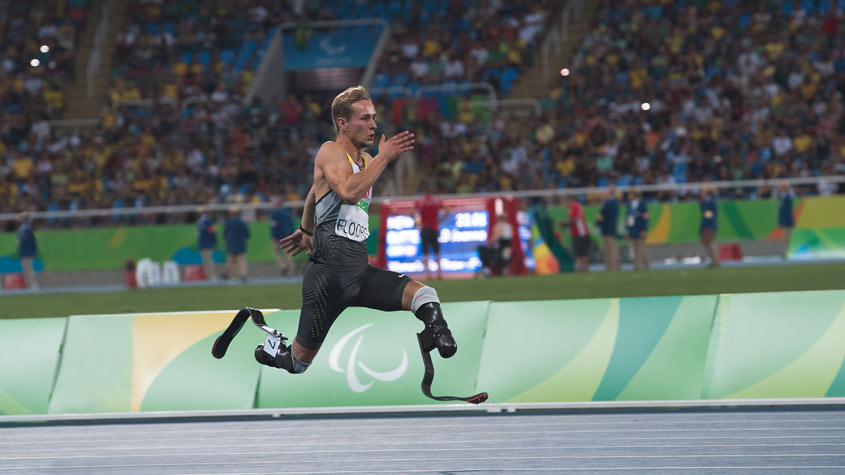This image depicts a man with prosthetic legs, often referred to as "blades," sprinting in a track race at a stadium. The man has blonde hair and is wearing a black, one-piece track suit that features a tank top design at the top and tight shorts at the bottom. His racing bib, marked with the name "FLOORS" in black text on a white background, is prominently displayed on his chest. The prosthetic legs are black and designed with high, flat bars that act as feet, both of which are off the ground, indicating he is in mid-stride. His arm muscles are prominently flexed as he exhibits a powerful sprinting motion. The track surface is gray, lined with white markings. There are officials in blue jackets and tan pants visible near the track, alongside green and yellow painted barriers, adding vibrancy to the scene. The stands are packed with spectators, suggesting this is a significant and well-attended sporting event, potentially a high-profile competition for athletes with disabilities.